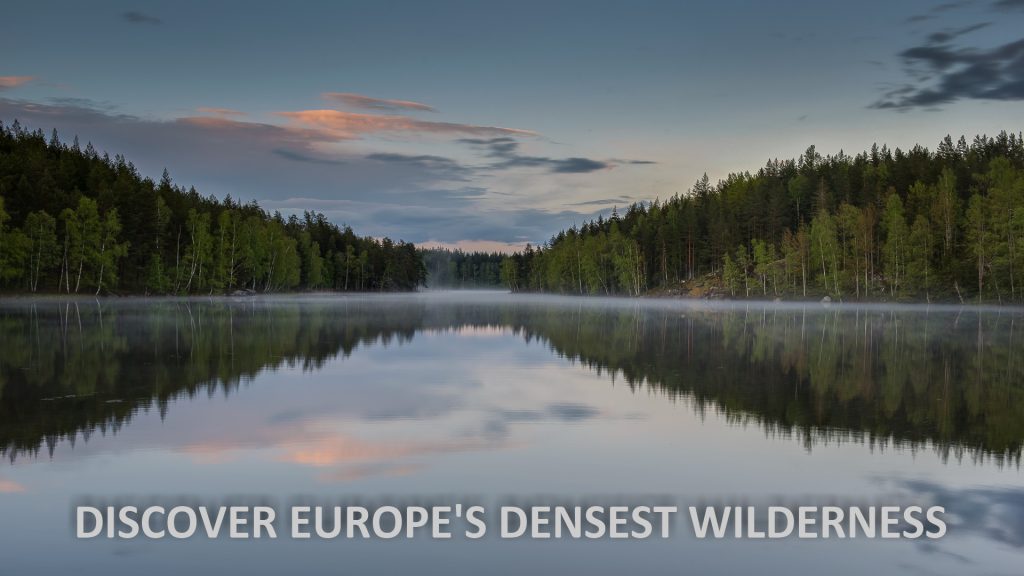The advertisement is a horizontal promotional poster for tourism in Europe, prominently showcasing the slogan "DISCOVER EUROPE'S DENSEST WILDERNESS" in white, capital letters at the bottom. The photograph captures an outdoor scene, featuring a high blue sky adorned with various cloud formations highlighted in whites, pinks, and darker grays, suggesting either sunrise or sunset. Dense forests of coniferous trees line both sides of a large, still body of water, likely a wide river. The water, reflecting the trees and the colorful sky, also harbors a slight layer of mist, adding to the serene atmosphere. The image appears to be taken from a vantage point in the middle of the river, possibly from a boat, and hints at the wilderness stretching far into the distance where the river either splits or transitions into a lake. The foreground suggests the onset of dusk, enhancing the tranquil and untouched beauty of Europe's densest wilderness.